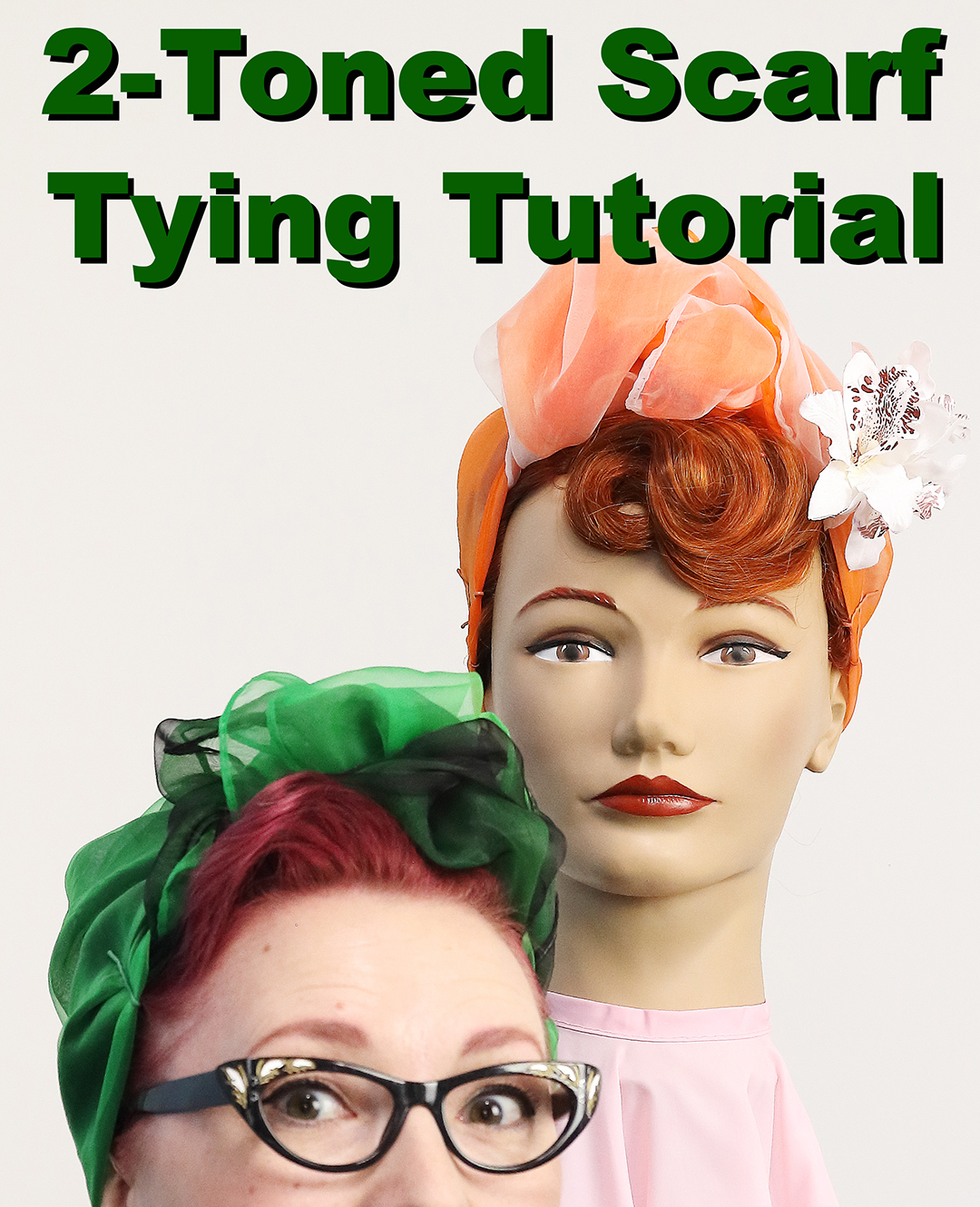This image serves as an advertisement for a two-tone scarf tying tutorial. In the foreground, the top half of a real woman's face is visible, adorned with black plastic-framed glasses that have gold and white details. She has dyed red hair tucked under a green scarf. In the background, a mannequin with similar red hair is shown wearing a peach-colored scarf embellished with a small white flower on the side. The mannequin's head is fully visible, complete with a pink fabric around the neck. The scene is clearly aimed at teaching viewers how to tie scarves, as indicated by the text "Two-Tone Scarf Tying Tutorial" prominently displayed at the top of the image. Both the real woman and the mannequin share a striking resemblance, which reinforces the instructional theme of the scarf-tying technique.